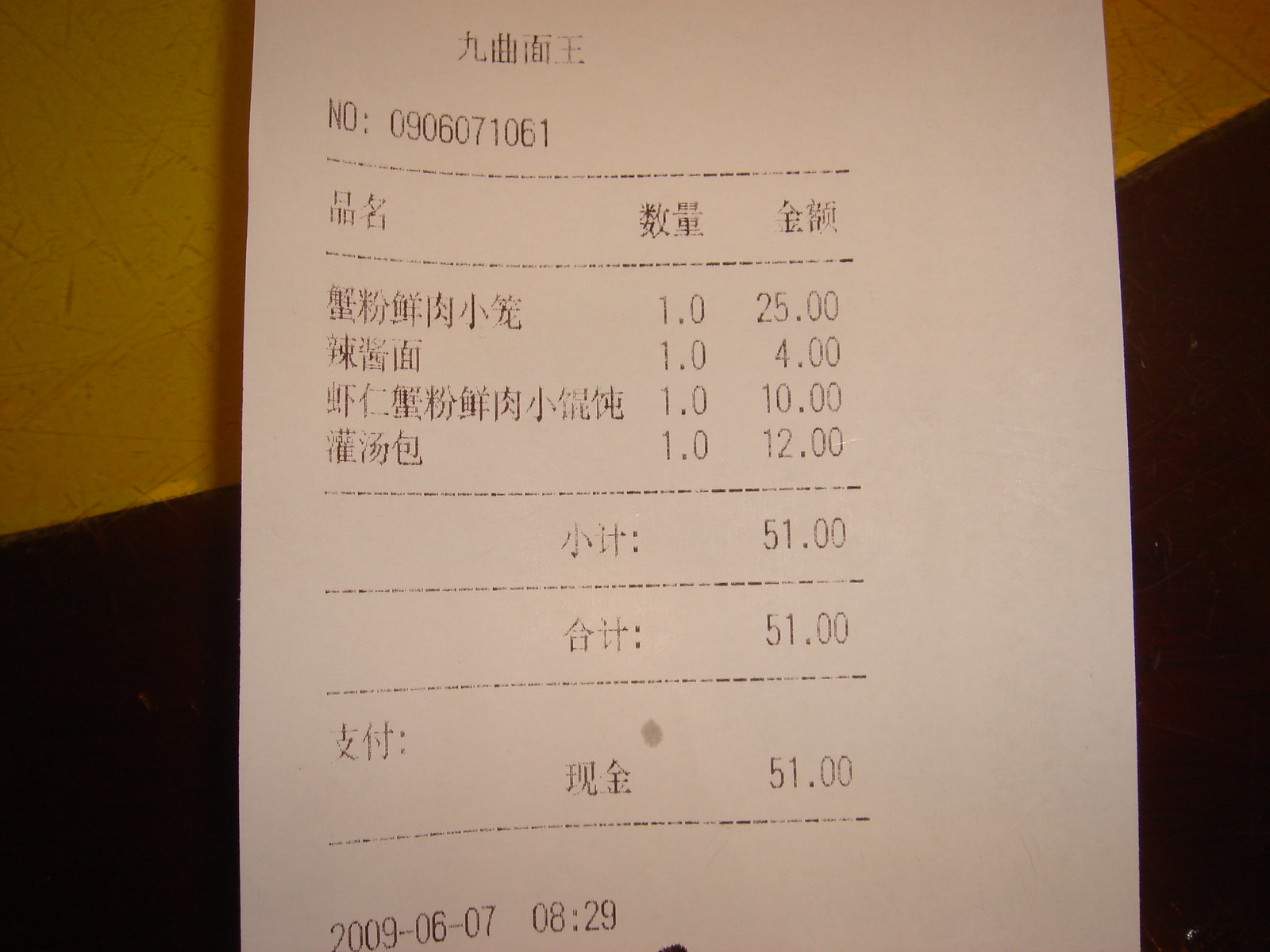This image displays a black and white receipt prominently featuring Asian characters, which suggests it is from an Asian country, though the exact language and currency are unspecified. The receipt lists several items with numerical values next to them. Specifically, the entries include: one item priced at 25, another at 4, a third item at 10, and a final item at 12. These amounts sum up to a total of 51 in the unidentified currency. Additionally, the receipt is dated June 7th, 2009, with the time recorded as 08:29.